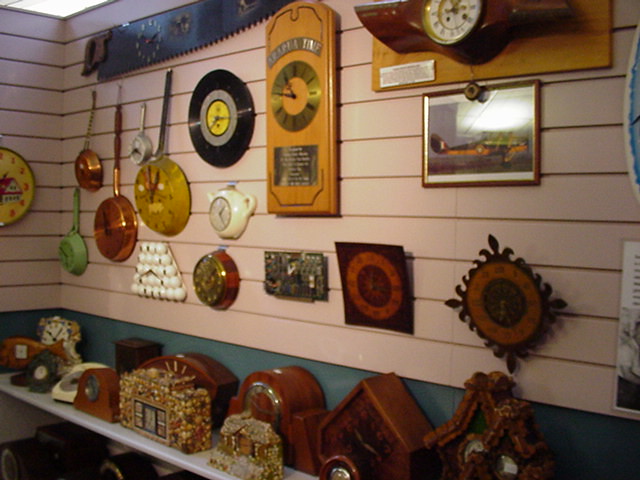The image depicts a corner wall in an antique shop, adorned with a captivating array of clocks. The wall itself is painted in light pink with horizontal stripes, accented by a dark blue border underneath. A white, almost marble-like shelf, filled with various clocks suitable for a bedroom stand, runs along the bottom of the display.

The clocks on the wall are creatively themed, showcasing the shop's eclectic taste. On the far left, five frying pans, three full-sized and two smaller decorative ones, have been ingeniously converted into clocks. Nearby, an old vinyl record and a long saw with a clock embedded in its metal blade add to the unique collection. A particularly striking piece features a large orange wood plaque with a traditional ornate clock mounted to it. Other wall-mounted clocks include ones shaped like a teacup, a circuit board, and a stack of either eyeballs or golf balls arranged in a pyramid. There is also a regular wooden clock with intricate designs and a shiny gold-framed clock for a touch of classic elegance.

On the white shelf below, a variety of clocks are arranged. Among them, there's a cottage-like clock made of what appears to be rocks or perhaps candy, and another bulky one with different face plates. A standout piece on this shelf is an old rotary dial telephone repurposed into a clock. Most of the shelf clocks are homogenous, predominantly made of dark woods, with two exceptions near the front, which are crafted from multicolored beads or circular objects.

In the arrangement, there's also a framed picture of an old-timey plane, adding a nostalgic touch. The overall setting, filled with both conventional and unusual timepieces, suggests a delightful journey through time and creativity.